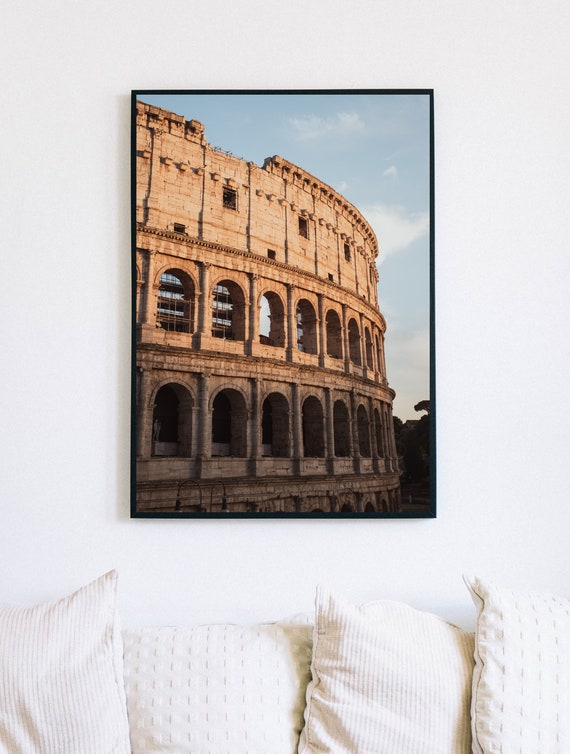The photograph, hanging on a white wall, captures a close-up section of the Roman Colosseum standing upright under a light blue sky dotted with white clouds. The Colosseum, in its characteristic tannish brown stone, basks in partial sunlight, casting half of the structure in shade. Surrounding the framed picture, which has a light black border, are four uniquely textured throw pillows arranged beneath it. The pillow on the far left features stripes, the next one displays raised markings, followed by another striped pillow, and the pillow on the far right also shows raised markings. The scene appears to be indoors, possibly in a living room or bedroom, with the setup resembling a cozy corner on the back of a couch.